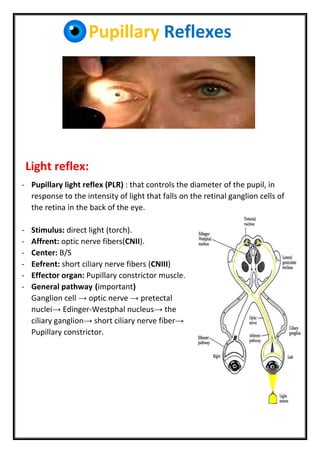This detailed chart, which appears to be from a health information website or medical book, educates viewers about pupillary reflexes. The content is framed in a black-bordered white rectangle, prominently titled "Pupillary Reflexes" at the top, alongside a blue eyeball logo. Below this title, there is a close-up color photograph of a light-skinned woman with light blue eyes. An ophthalmologist or optometrist is shining a light into her right eye, causing its pupil to constrict, while her left eye shows a normal-sized pupil. The patient's right eyelid is held open by a finger.

Underneath the photograph, the text explains the concept of the "Light Reflex." This "Pupillary Light Reflex (PLR)" controls the diameter of the pupil in response to light intensity hitting the retinal ganglion cells at the back of the eye. Key terms are broken down with explanations in bullet points, such as the stimulus (direct light or torch), afferent pathways (optic nerve fibers), the central processing area (brain stem or BS), efferent pathways (short ciliary nerve fibers), and the effector organ (pupillary constrictor muscle). 

The chart also details the general pathway of the reflex, stating: ganglion cell leads to the optic nerve, which leads to the pre-tectal nuclei, then to the Edinger-Westphal nucleus, followed by the ciliary ganglion, short ciliary nerve fibers, and finally the pupillary constrictor muscle. To the right of this explanation is a detailed, top-down anatomical diagram illustrating the connection between the eyes and various brain structures. This diagram labels and visually traces the pathway described, enhancing the educational value of the chart.